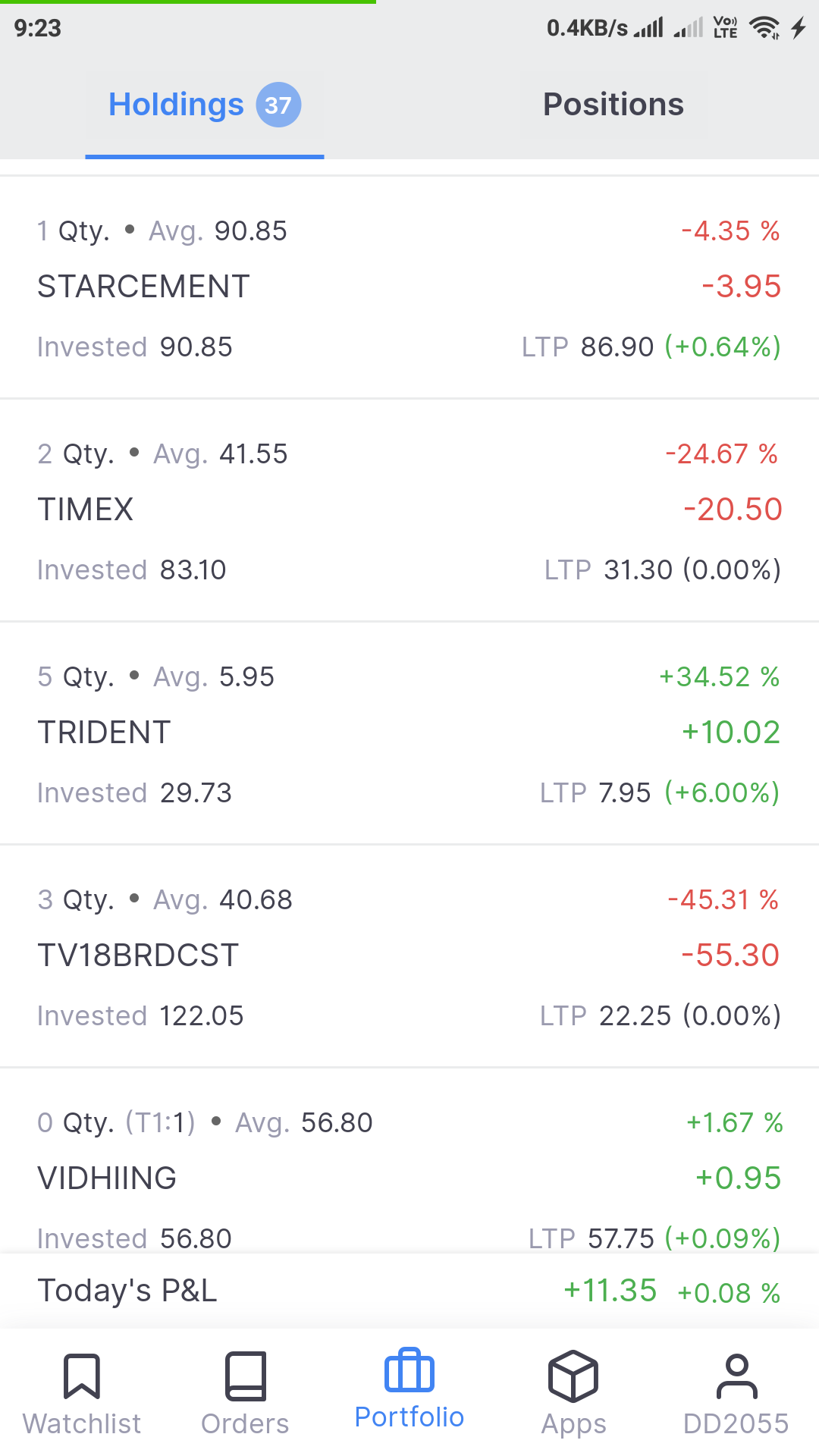In this screenshot of a mobile device, the display vividly shows various crucial details. At the top left corner of the screen, the time is prominently displayed, reading 9:23. Shifting your gaze to the top right, a multitude of status indicators can be observed. The mobile connection speed icon is present alongside the Wi-Fi signal strength, which is at its maximum with all four bars illuminated. Additionally, a lightning bolt symbol signifies that the phone is currently charging.

Focusing on the screen's content, you are presented with two main categories: "Holdings" and "Positions." The interface lists five specific items within these categories, suggesting a detailed overview of different assets or stocks the user holds. 

Towards the bottom of the screen, a navigation bar is visible, facilitating quick access to various features of the application. The bar includes labeled tabs: "Watchlists," "Orders," "Portfolio," and "Apps," allowing the user to seamlessly switch between different sections of the app for a comprehensive financial management experience.